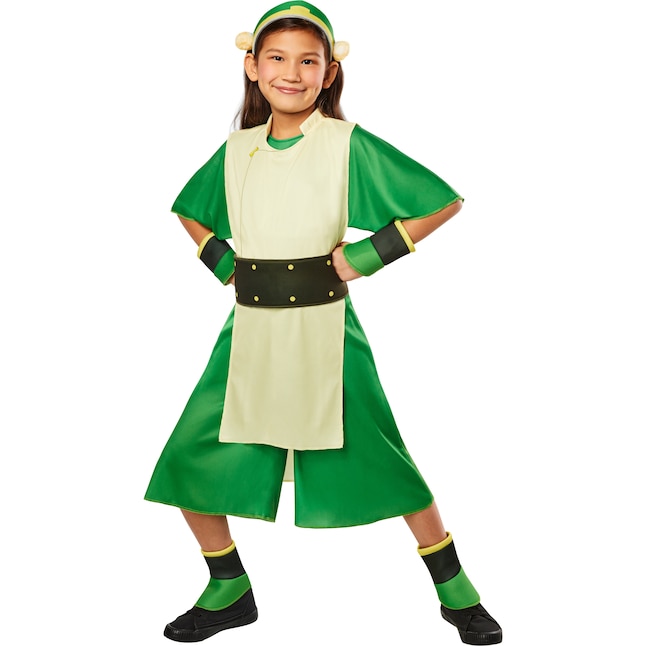The image is of a young girl, around 10 years old, dressed as Toph from the animated TV show "Avatar: The Last Airbender." She is striking a confident action pose with her legs apart and hands on her hips, standing at an angle. She has long brown hair and a tan skin tone, complemented by an outfit rich in greens and accented with various other colors. Her costume features an emerald green tunic with sleeves reaching her elbows and pant legs in a culotte style that ends just below the knee. Over this, she wears a pale khaki-colored, almost white, apron-like robe that covers the front. 

Her outfit is adorned with a wide black belt around her waist, which is decorated with yellow buttons. She also wears black shoes with green, black, and yellow spats covering her ankles, matching the wristbands of the same colors. On her head, she has a green headband featuring two white bulbs that resemble ears, enhancing her resemblance to the character. She is smiling brightly, clearly enjoying her role-play as Toph, emanating a strong and happy presence against the white background.